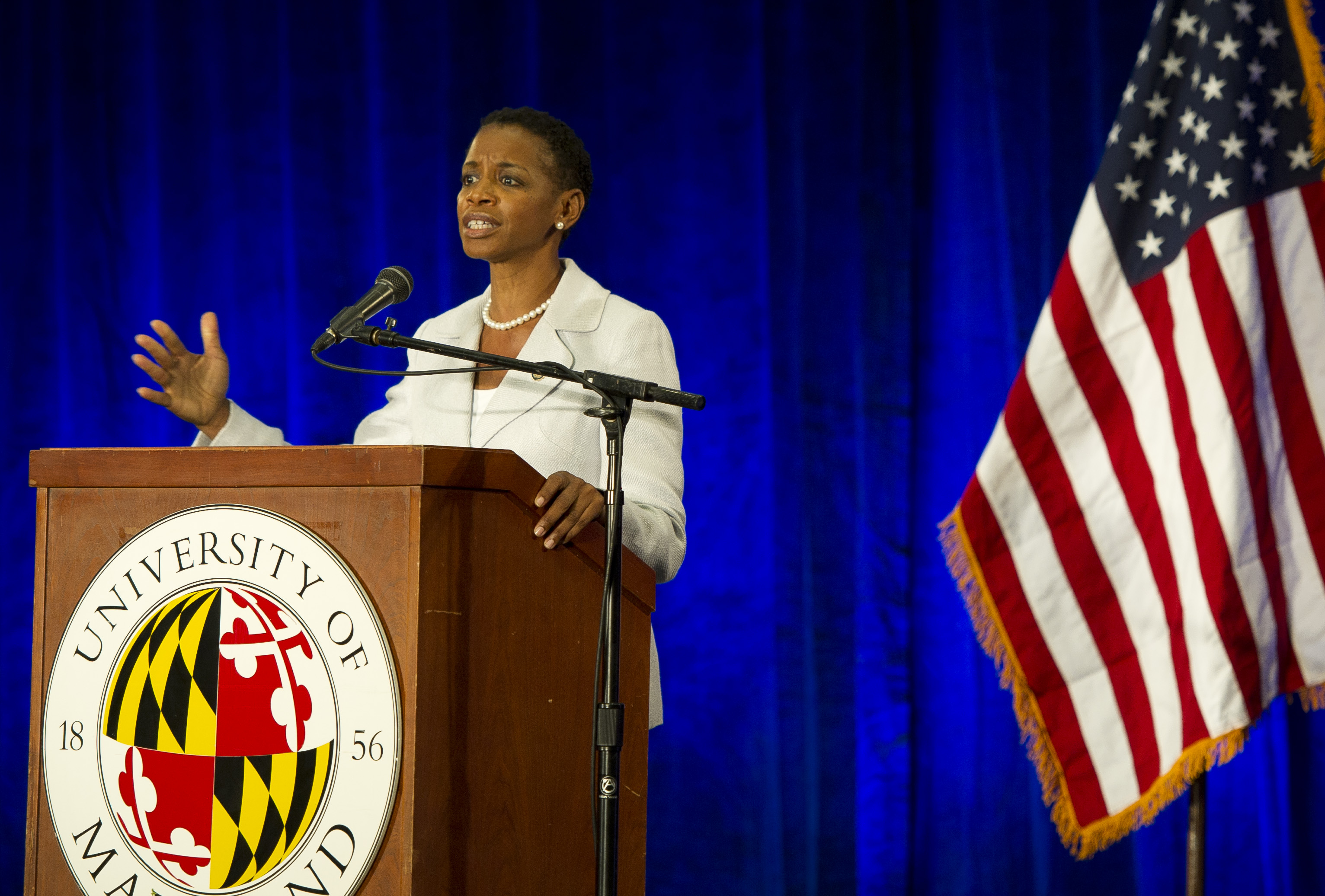The photograph captures an African-American woman with very short, close-shaven hair, likely standing in a lecture or presentation setting at the University of Maryland. She is immaculately dressed in a cream-colored suit jacket over a white undershirt, accessorized with white pearl earrings and a matching pearl necklace. The backdrop features a dark blue curtain, and to her right, a prominently displayed American flag adds a touch of formality to the scene.

She stands confidently at a large, well-worn, dark brown wooden podium. This podium is adorned with a distinctive white circular logo, which features the text "University of Maryland" in a serif font, alongside its founding year, 1856, split by a globe-like emblem with red, yellow, black, and white accents. A microphone atop a stand is positioned before her, suggesting she is engaged in delivering a speech or presentation. The setting within the building emphasizes the academic and institutional atmosphere of the University of Maryland.